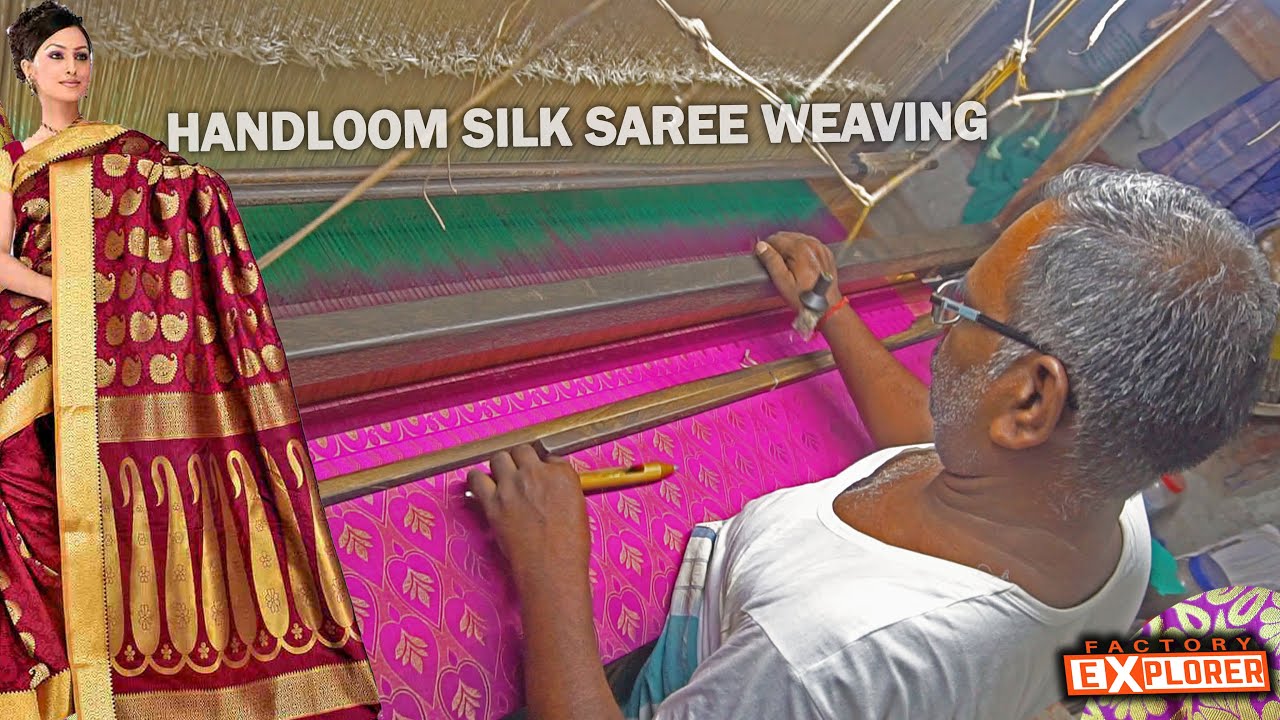The image is an overhead, slightly downwards, view capturing a traditional scene of silk sari weaving. On the right side, a man with gray hair and glasses, dressed in a white shirt, is focused on his work at a loom. He is weaving intricate gold flower designs into a section of purple fabric. His hands are stretched out in front of him, actively engaged, and he holds a pencil in his left hand. To the left of the image, a woman dressed in a stunning red sari adorned with gold trim and elaborate etchings stands with her face turned towards the camera. Her dark hair is wrapped elegantly around her head, and her right arm extends down beneath the fabric draped around her. Above the loom, gold designs add a touch of elegance to the scene. A large glass piece with metal trim is visible towards the front, and brown thread stretches across the top of the image. In the bottom right corner, "Factory Explorer" is prominently displayed, where the word 'Factory' is in orange text on a black background, and 'Explorer' features orange text on a white background, except for the 'X,' which is in white text on an orange background. The title at the top reads "Hand Loom Silk Sari Weaving," indicating the traditional and artisanal nature of the process.